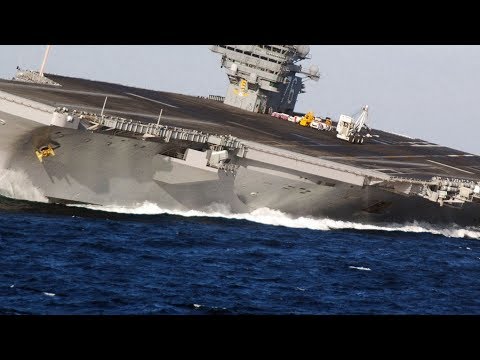The image captures a large, gray aircraft carrier navigating in the deep blue ocean, with dark navy waves creating tufts of white foam as they collide with the vessel. The aircraft carrier, which is massive in scale, appears to be leaning heavily to one side, possibly due to the dynamic motion of the ocean waves. The top deck is flat and reminiscent of a roadway, paved with white lines for aircraft operations. Toward the back left of the vessel stands a multi-storied gray tower adorned with rows of windows and numerous antennas. Nearby, several strapped-down vehicles and a securely fastened crane are visible on the deck. The bottom of the aircraft carrier displays a slimmer profile compared to its broader top. The dramatic scene is highlighted by the black borders at the top and bottom of the image, giving it a cinematic feel.